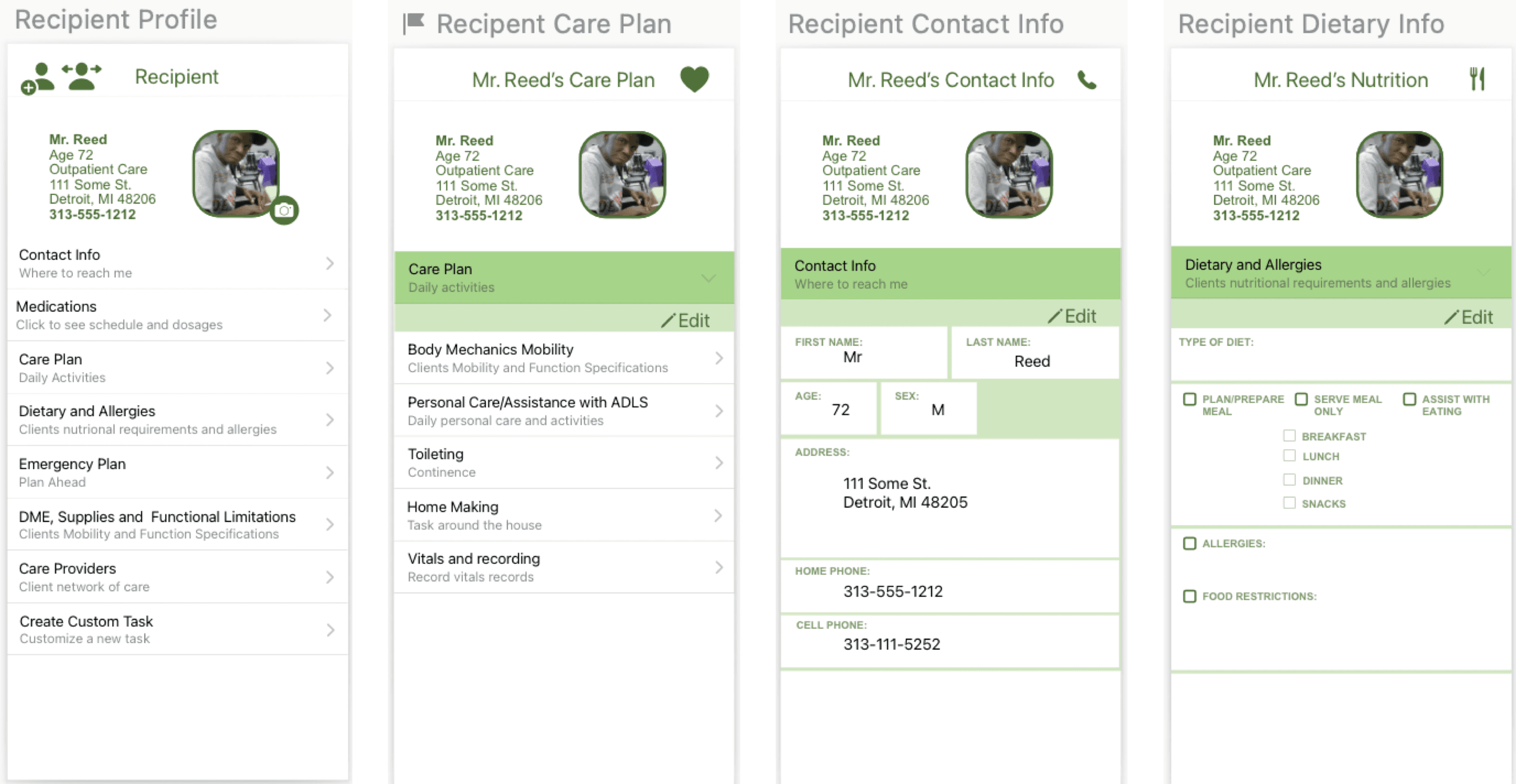The image depicts a structured, vertical arrangement of four distinct forms, all containing information about the same individual. These forms are titled as follows, from left to right: "Recipient Profile," "Recipient Care Plan," "Recipient Contact Info," and "Recipient Dietary Info." Each form features green text consolidating various details about the recipient, Mr. Reed, a 72-year-old outpatient. His address is listed as 111 Some Street, Detroit, Michigan 48206, and his phone number is 313-555-1212. The forms collectively provide comprehensive information to ensure Mr. Reed's proper care, encompassing his personal details, healthcare requirements, contact information, and dietary needs. This well-organized, multi-tab layout facilitates easy reference and efficient care management.